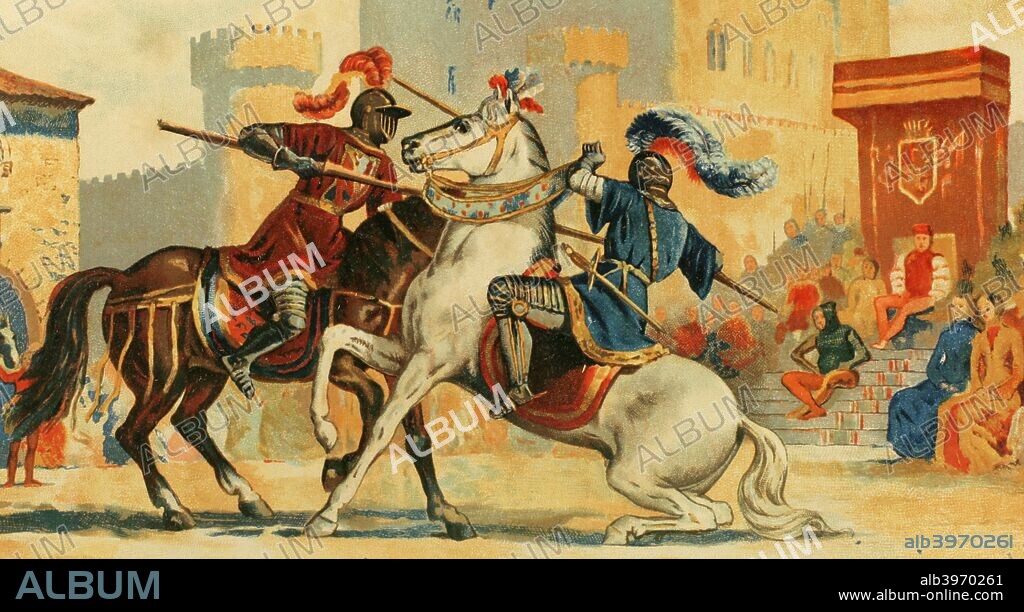The image is an album cover titled *Medieval Horses Buried in London*. The scene illustrates a dramatic jousting match between two knights on horseback, set against the backdrop of an imposing stone castle. The bleachers are filled with spectators watching intently. A knight in red armor, complete with a red feathered helmet, is mounted on a tan horse and appears to be gaining the upper hand. His lance is striking a knight in blue armor, who also dons a blue feathered helmet and is precariously balanced on a white horse that is struggling on its haunches. The blue knight, with a sword hanging by his waist, seems to be in peril as the red knight's lance makes contact. Across the image, white and semi-transparent gray text spells out "ALBUM." The bottom of the image features a black border with gray letters spelling "ALBUM" on the left side and the small white text "ALB3970261" adjacent to "www.album-online.com" on the right side.